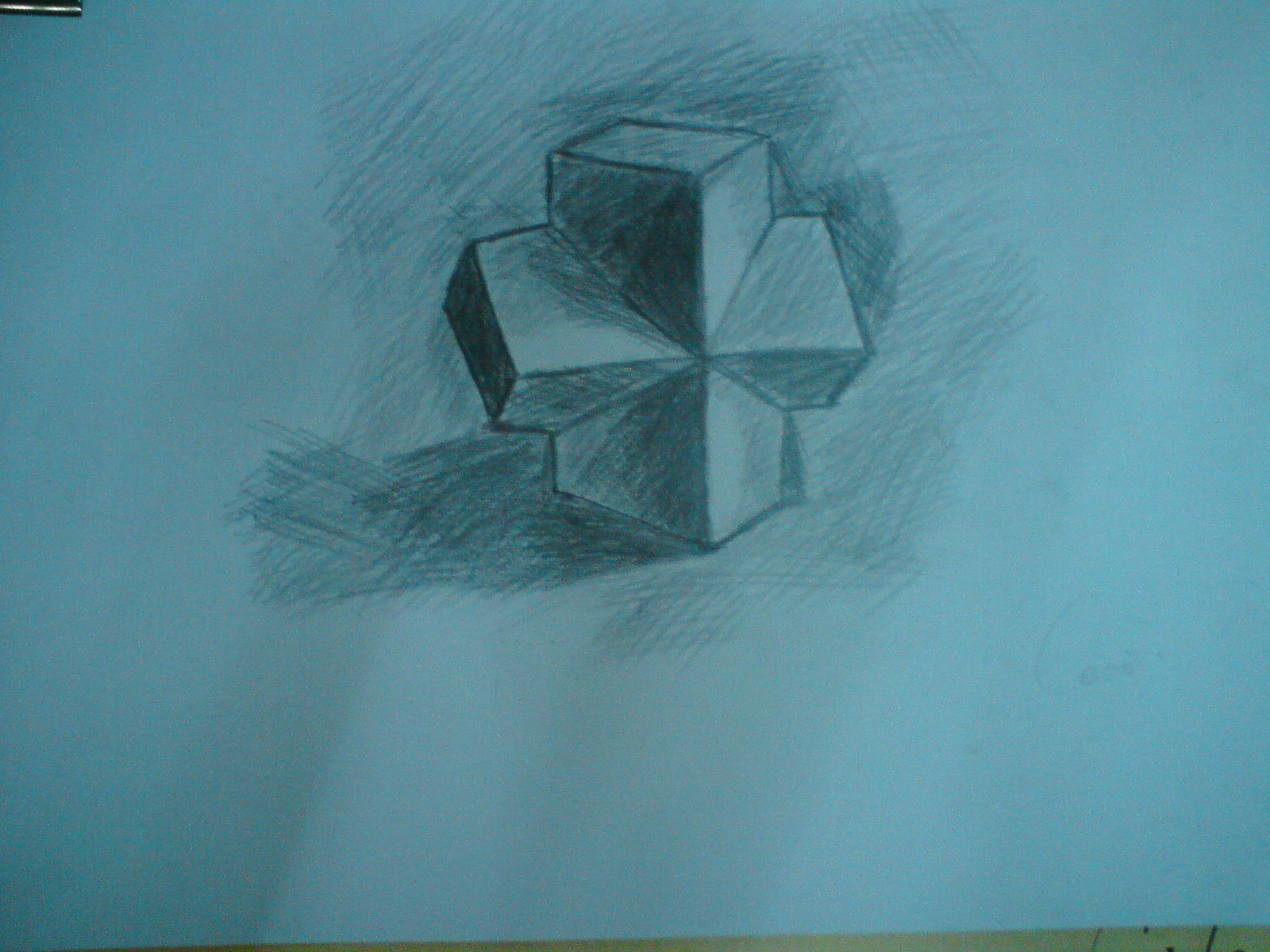The drawing on light blue paper showcases a meticulously detailed pencil sketch of two intersecting rectangular prisms positioned upright. The first rectangular prism is drawn to emphasize its three-dimensional form. It features a lighter top side and a light right side, whereas the front and left-facing sides are shaded in a darker tone to enhance its depth and perspective.

Intersecting the first prism in the center is a second rectangular prism extending horizontally. The top section of this intersecting prism, slightly tilted towards the viewer, is lighter in shading. The left end of this horizontal block is the darkest shaded area in the drawing, creating a strong contrast. The underside and front of this second block are shaded with intermediate tones.

The artist also skillfully added shading around the structures to emphasize their placement and the direction of light. There is subtle shading on the paper to the left of the prisms, a bit above them, and to the right and underneath them, using varying tones to reflect the shadows cast by the intersecting blocks.